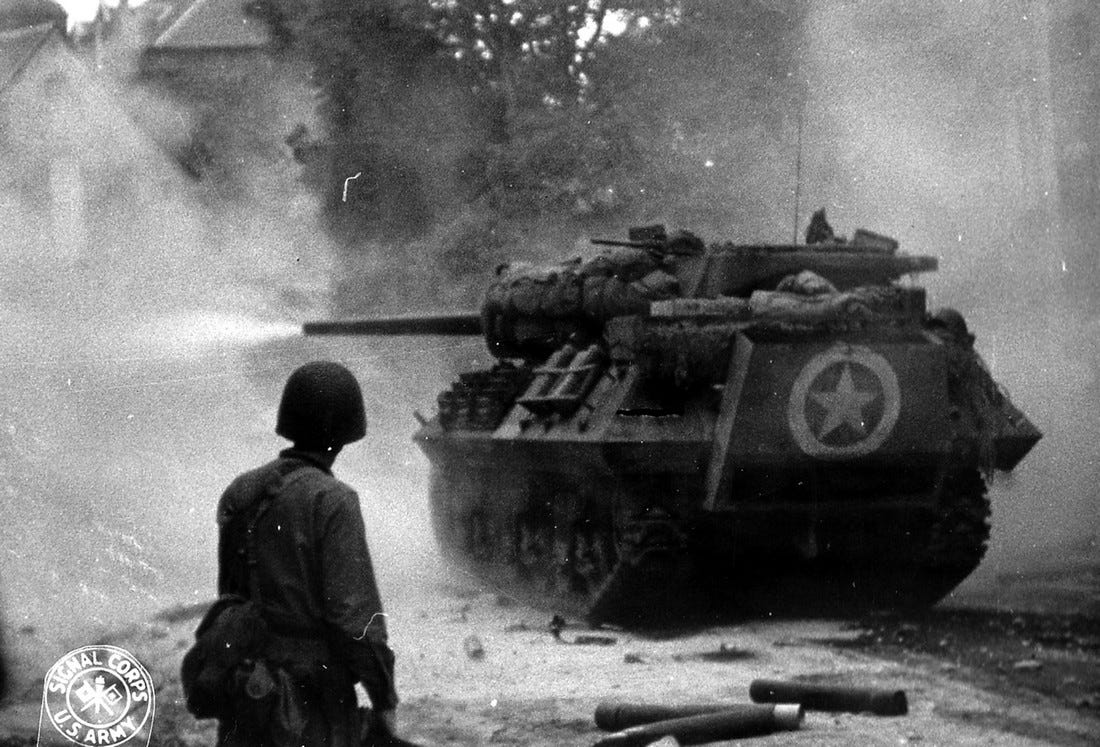This evocative grayscale wartime photograph captures a moment during World War II, depicting a U.S. Army tank actively engaged in a military operation within what appears to be a residential setting. The tank, distinguished by its sloped armor and adorned with infantry equipment strapped to its sides and back, prominently features a white star with a circular border on its engine block. Positioned to the left and rear of the tank is a soldier, clad in standard army gear including a metal helmet and utility packs, intently observing the action. The tank is firing its cannon towards a target on the left, with smoke and light emanating from the barrel, indicative of a recent discharge. The street shows evidence of heavy engagement with spent cannon shells scattered about. In the background, eaved buildings and a forest can be discerned, adding depth to the scene. At the bottom-left corner of the photograph, the emblem of the Signal Corps U.S. Army is displayed, featuring two crossing flags over a torch-like object, underscoring the photo's military context.